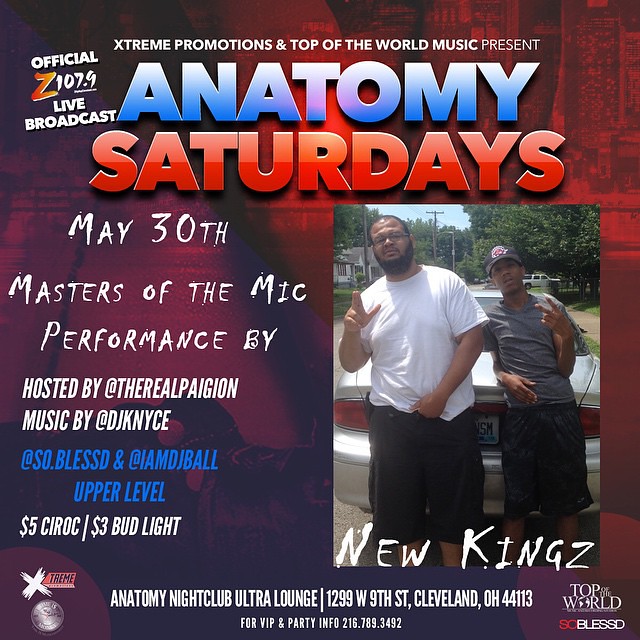This image features an advertisement for the "Masters of the Mic" event, scheduled for May 30th, presented by Extreme Promotions and Top of the World Music, hosted by The Real Pageon with music by DJ KNYCE. The official Z107.9 live broadcast will take place at Anatomy Nightclub Ultra Lounge, located at 1299 West 9th Street, Cleveland, Ohio, 44113. The flyer prominently displays additional details, including drink specials: $5 Ciroc and $3 Bud Light, alongside contact information for VIP and party inquiries: 216-789-3492.

The background of the flyer is a maroon and burgundy gradient, creating a vibrant and dynamic look. The top section highlights "Extreme Promotions and Top of the World Music Present," followed by "Anatomy Saturdays" in bright blue and red caps. Just below, it mentions "Masters of the Mic" in white text.

To the right, there's a photograph of two African-American men standing against a white car. One, wearing a white t-shirt and black shorts, displays a hand sign. The other, in a gray t-shirt, black shorts, and a black baseball hat, also displays hand symbols. Both men are positioned below the text "New Kings."

The flyer also includes several noteworthy logos and social media handles: @SO.Blessed and @IMDJBall, emphasized in white and red. Additionally, there is a logo for Top of the World, featuring an earth symbol replacing the "O," and another for Extreme Promotions with a stylized "X."

Every detail, from social media tags and drink specials to meticulous event information, ensures that this flyer effectively communicates the excitement and exclusivity of the upcoming event.